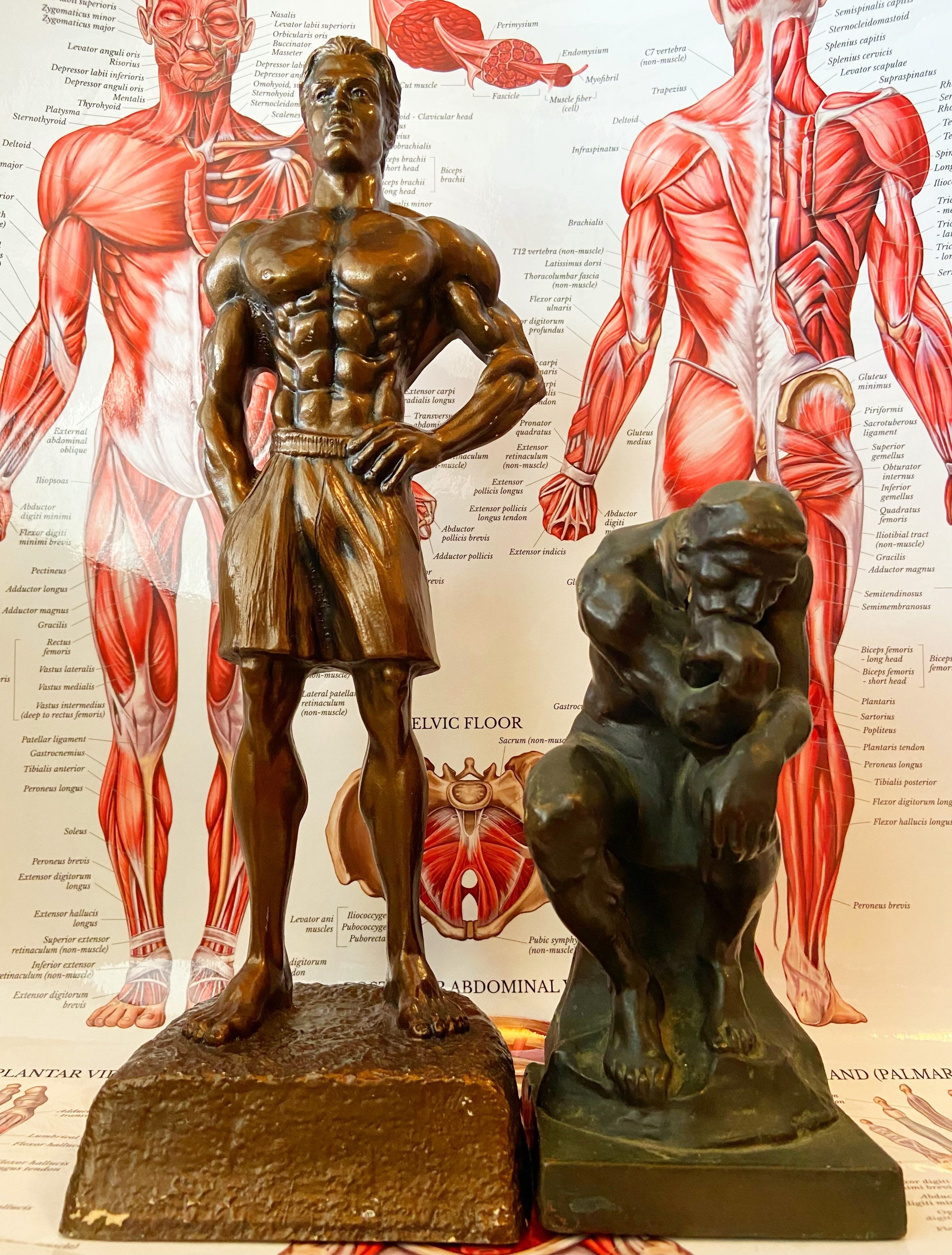In this photograph, two prominently detailed bronze statues are positioned in front of a large anatomical chart that vividly illustrates the muscular structure of the human body, both front and back. The chart covers much of the wall behind the statues, adding a rich educational backdrop to the scene. The photograph itself is twice as long on the sides as it is tall.

On the left, there is a statue of a muscular man standing confidently on a square base, which shows white coloring beneath where the bronze has chipped away. He is bare-chested, wearing only shorts, and his sculpted physique is displayed prominently. His stance exudes confidence with his right hand in his pocket, and the remaining hand resting on his waist, his chest pushed out, and his gaze fixed straight ahead.

To the right, the second statue depicts a man in a contemplative pose, seated and leaning forward with one hand resting on his chin, and his elbow supported by his knee, embodying the traditional "The Thinker" posture. This statue, like the first, has a dark greenish-bronze patina. The detailed portrayal of muscles in both statues resonates with the anatomical chart behind them, where the muscles are depicted in red, providing an apt backdrop that highlights the theme of human musculature and physical strength in art.